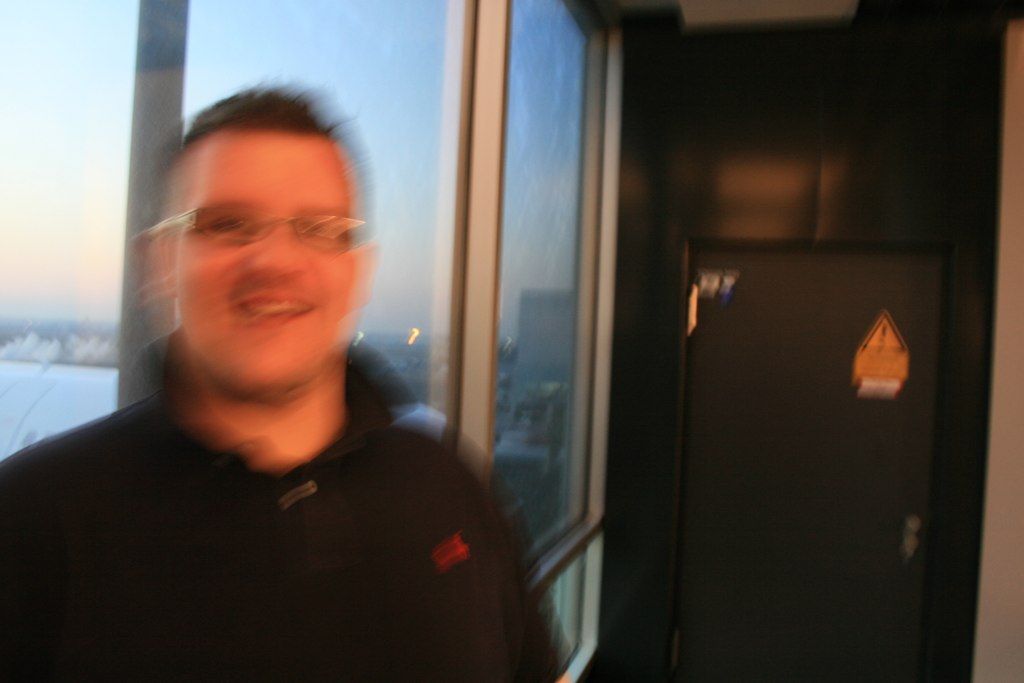A highly blurred and underexposed photograph depicts a man with a mustache, large chin, and wire-rimmed glasses smiling as he stands in an indeterminate indoor location. He wears a black polo shirt or jacket with the collar turned up and a small, red logo on the chest. His hair is closely cropped on the sides with a mullet on top. He stands in front of large aluminum-framed windows that appear to be in a high-rise office building, possibly overlooking a body of water, with a blue evening sky and distant buildings visible through the glass. To the right of the picture is a dark cabinet or safe with a yellow warning label.